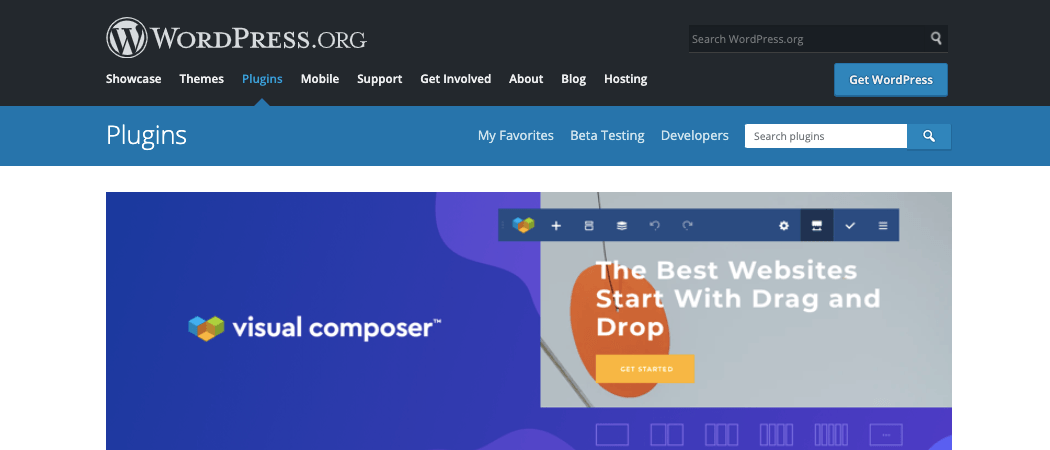The top navigation area of the WordPress website includes options for Showcase, Themes, Plugins, Mobile Support, Get Involved, About, Blog, and Hosting. A search bar and a prominent blue "Get WordPress" button are also visible. The main banner is black with the text "WordPress" in white, creating a striking contrast.

The user has navigated to the "Plugins" section, which is followed by options for "My Favorites," "Beta Testing," "Developers," and another dedicated search bar for plugins. Below, there's a graphic banner for a visual composer plugin. The banner features a tagline, "The best websites start with drag and drop," along with a visual preview of the plugin in use. The preview showcases a three-dimensional, cube-like interface that vaguely resembles a heart and is presented at an angle. There is also an orange "Get Started" button on this banner. The main website background is white, while the background of the banner graphic itself is blue.